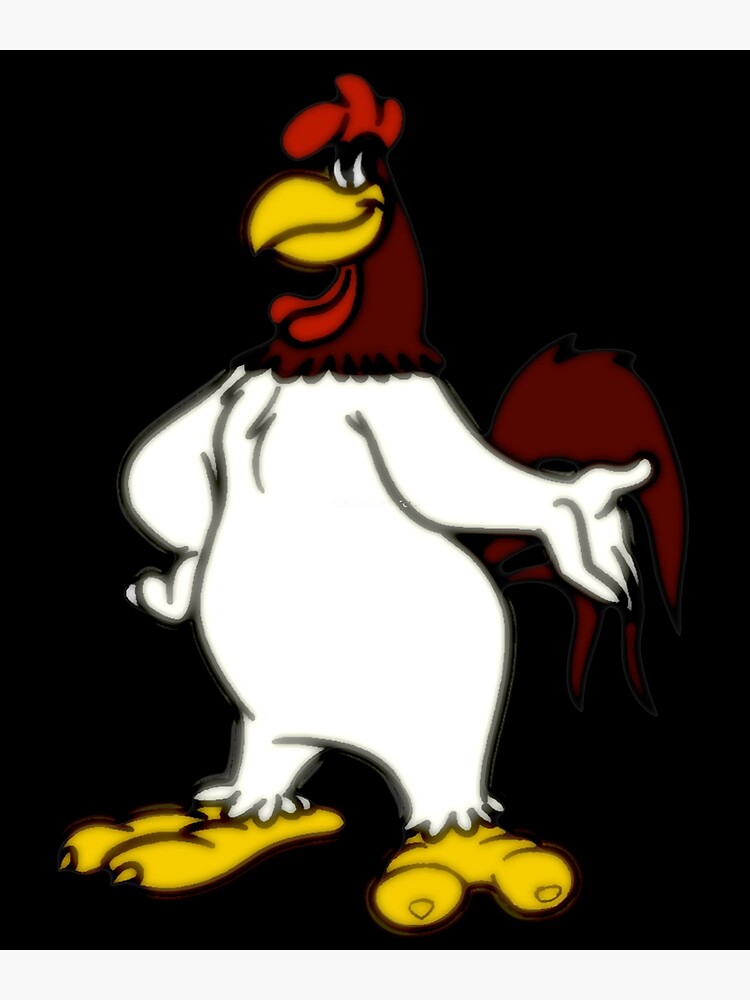This vertical rectangular cartoon image features Foghorn Leghorn, the confident and iconic rooster from mid-20th-century cartoons. The character stands out prominently against a very dark, black background, with a subtle reddish area revealing an outline of some structure. Foghorn Leghorn, a large rooster, has a white plump body with striking yellow feet and a yellow beak. His head, upper neck, and pronounced wattles under his chin are a vivid red. He has large, expressive eyes that look off to the side, conveying a confident demeanor. His left arm is stretched out, palm open and thumb up, as if he's making an emphatic point, while his right arm rests on his hip. His dark red tail is partially visible, curving behind his hand. This image, resembling neon artwork, captures Foghorn Leghorn's bold stance and charismatic presence.